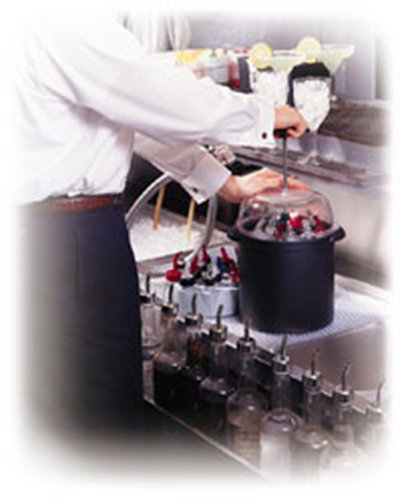In a portrait-oriented color photo with a feathered white edge, we observe a bartender immersed in his task. Positioned on the left side of the image, he is seen from the shoulders down, clad in a formal white shirt with dark buttons on the cuffs, a brown leather belt, and dark navy blue pants. His hands are engaged with a black hand-cranked ice cream making machine that features a clear top with a pump handle. In front of him on the counter lies a row of pouring bottles filled with various flavored syrups. To the left of the counter is an ice bin, while to the right, behind the bottles, sits a stainless sink and a counter. On the bar behind him are two margarita glasses garnished with yellow lemons. The overall scene is set in a restaurant or bar, where he appears to be preparing a dessert or perhaps a specialty cocktail.